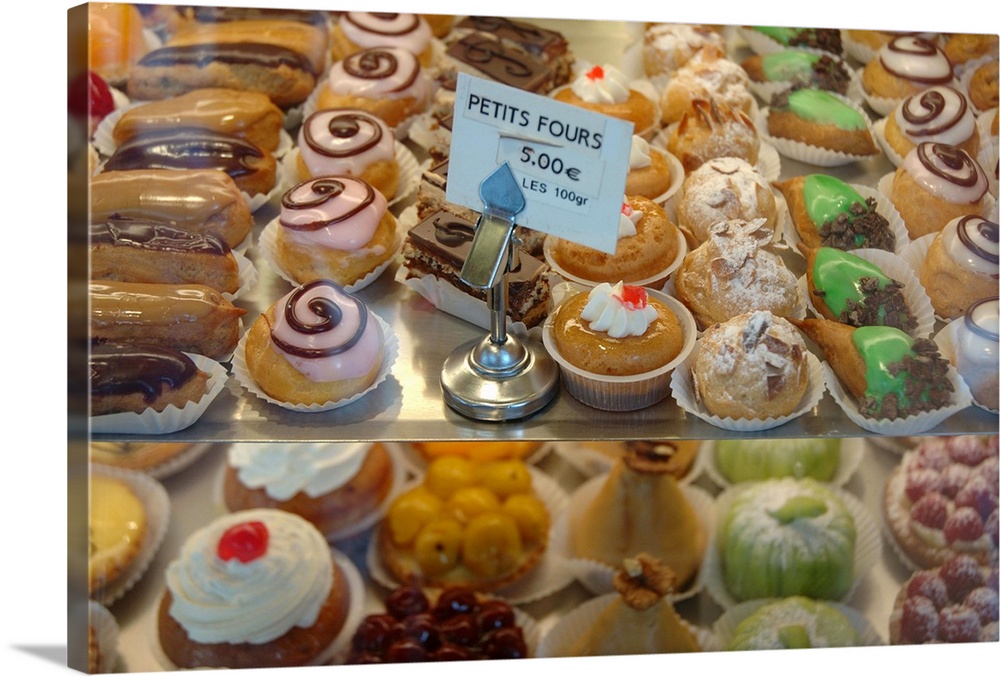This full-color, horizontally rectangular photograph is taken indoors using artificial lighting. The image showcases a display case of various pastries and desserts, all tempting and meticulously arranged in rows on two glass shelves. The backdrop is somewhat neutral, with a slight shadow visible at the bottom lower left, giving depth to the picture. On the middle shelf, a silver card holder holds a blue sign that reads "Petits Fours: 5 Euros / 100g," indicating this is likely a French-speaking store. The assortment includes treats such as eclairs, donuts, and other pastries adorned with different toppings—some with frosting, some with white or green cream, and others with glazes. The desserts range in colors and types, featuring a delectable variety that promises a high calorie and sugar content, making them look irresistibly delicious.